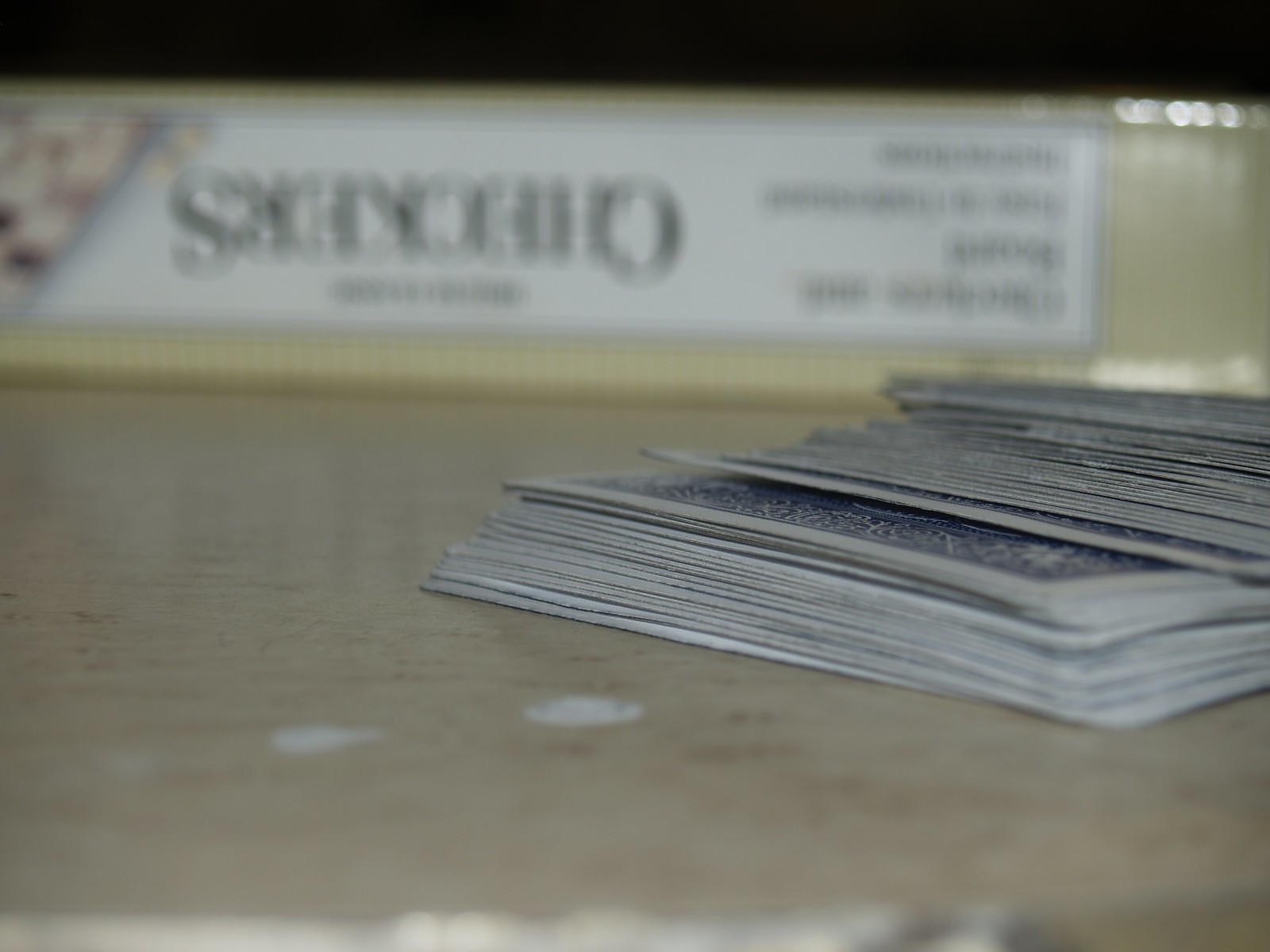This detailed landscape-style image portrays a weathered deck of cards positioned towards the right side of the frame. The stack of cards is arranged such that the top half leans backward while the bottom half lies flat against the glossy surface. The worn cards, displaying a blue pattern on their backs, suggest their age and usage over time. 

In the background, a sign with a cream-colored backdrop and white central section bears upside-down, black capitalized text, though the words remain indistinct due to blurriness. This sign features four lines of text on its right side, similarly unreadable but consistently black in color. 

The setting is completed by a grayish cream-colored surface beneath the cards and the sign, noted for its shiny, reflective quality that hints at an epoxy-like finish, adding a subtle sheen to the overall composition.